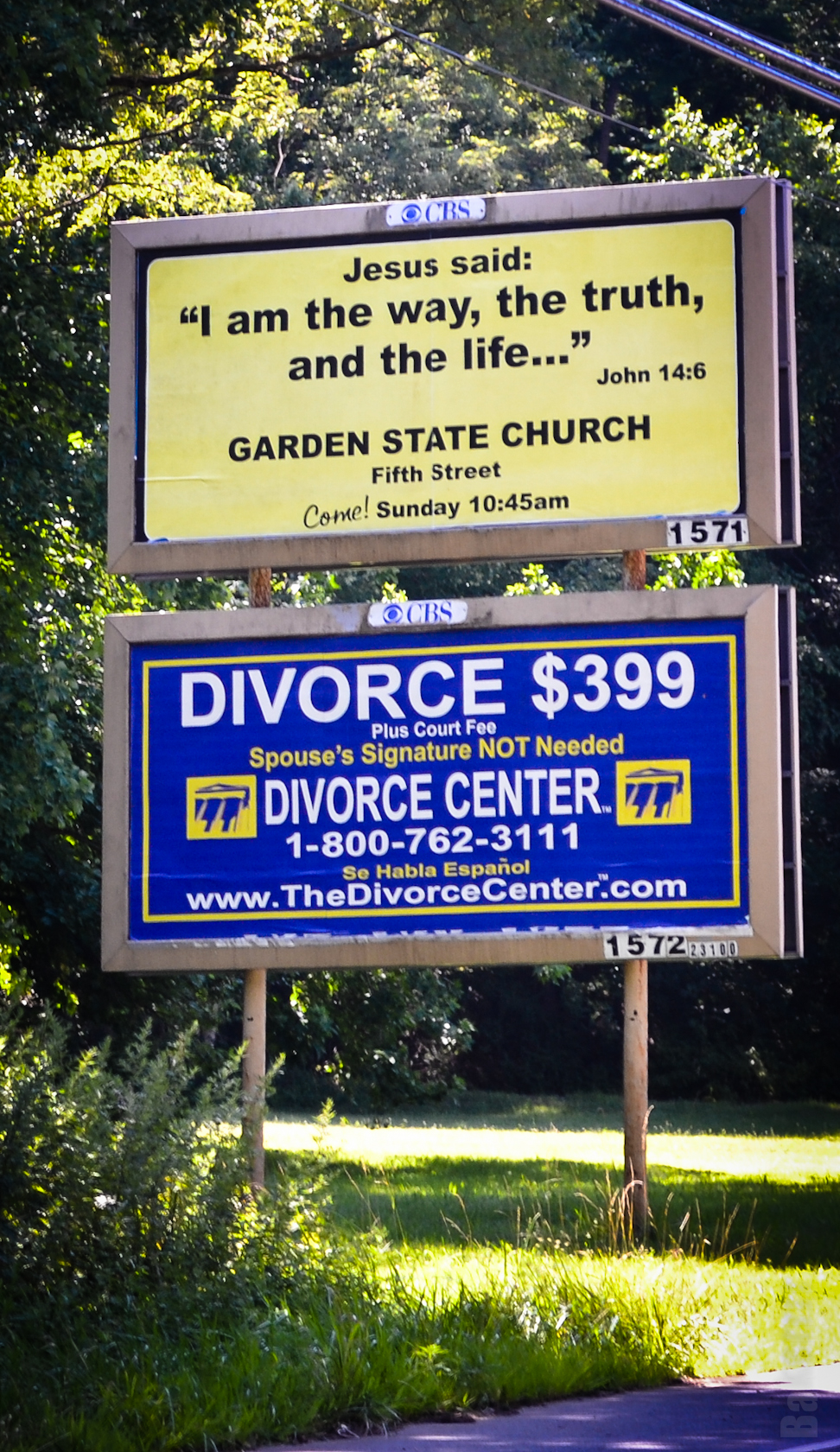Situated near a wooded roadside, two distinct signs are mounted together on rustic wooden posts, framed by a double-edged wood border. The top sign, featuring a white background and black text, carries a religious message and details: "Jesus says, 'I am the way, the truth, and the life.' John 14:6. Garden State Church, 5th Street. Come Sunday, 10:45 AM." Additionally, it includes the numbers "1571" and "1572," as well as "CBS."

Beneath this, a blue sign with white and yellow lettering advertises legal services, stating: "Divorce, $399 plus court fees. Spouse's signature not needed. Divorce Center, 1-800-762-3111. Se habla español. www.thedivorcecenter.com."

The juxtaposition of the religious and legal advertisements on traditional, non-digital signage provides a curious and somewhat humorous visual contrast.